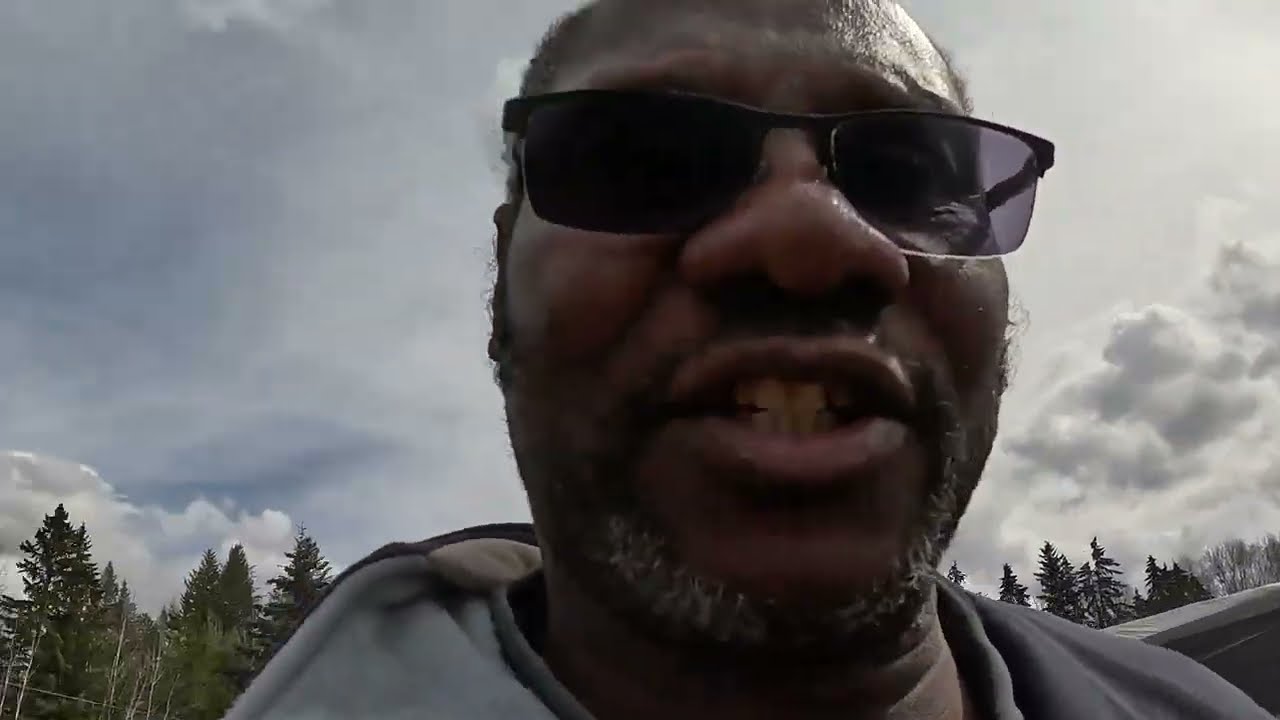The image is an up-close photograph of an African American man, possibly taken as a selfie or by someone else. The man is wearing black-rimmed sunglasses with a purple tint and no rim underneath the lenses. His short hair, sprinkled with gray, appears a bit squirrelly. He has a salt-and-pepper goatee, blending black and gray, and his mouth is open, showing his teeth under a slight shadow, with the middle two being the most visible. He sports a jacket that's white in the center with gray on the sides, resembling a gray hoodie. The background features a cloudy sky with varying densities of storm clouds, creating a dynamic circular movement effect in the backdrop. Flanking him on either side are pine trees with trunks that look somewhat balding and display shades of green from dark hunter to vibrant light green. In the image's bottom right corner, a concrete barrier extends behind the man’s shoulder, adding an additional layer to the backdrop's wooded landscape.